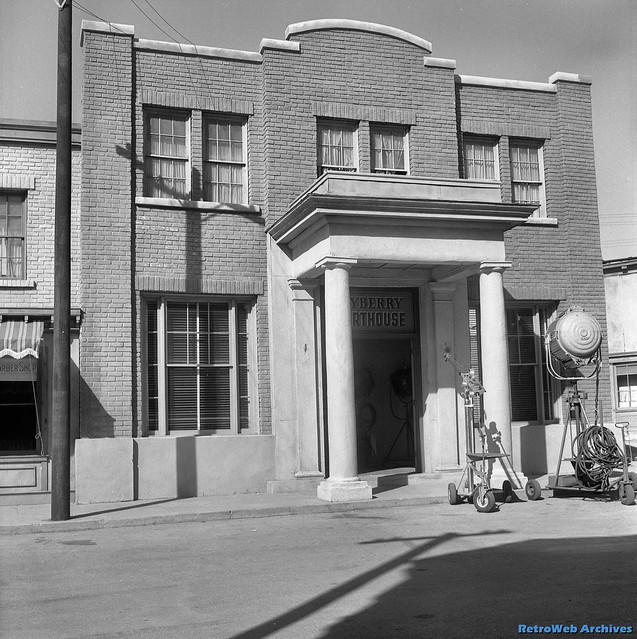This black and white photograph appears to depict the front of a courthouse building, likely the "Mayberry Courthouse" as suggested by the partial sign visible in the image, which reads "Y-B-E-R-Y" and "R-T-H-O-U-S-E". The building is constructed of brick, with two floors featuring windows; the lower floor has a central doorway flanked by windows, while the upper floor has three sets of windows. Above the doorway, two white pillars support a small roof. To the far left of the image, there is a tall wooden pole with power lines. Adjacent to the courthouse on the left, another structure with an awning is partially visible. On the right side of the image, beyond the courthouse, additional buildings are seen. The scene includes production equipment such as large lights and a camera dolly, indicating this could be a set photo, possibly from "The Andy Griffith Show." In the bottom right corner, the text "Retro Web Archives" is visible, suggesting the image is part of a digital historical collection. The sky above is gray, enhancing the vintage atmosphere of the photo.